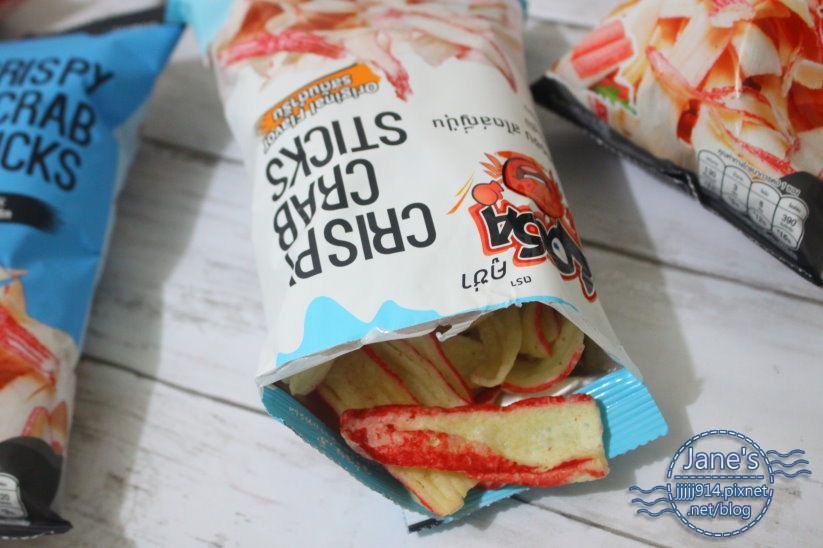This is a close-up color photograph of three bags of snacks positioned on a white wooden table made of horizontal wooden panels. The focal point is a centrally placed, upside-down, and opened white bag with a blue top, revealing its contents: crispy crab sticks, which are long, finger-shaped snacks with a golden color and red edges to resemble crab meat. The words "Crispy Crab Sticks" are visible in black but appear upside down due to the bag's orientation. Adjacent to this bag, partial views of two other bags can be seen; one has a blue edge, while the other is black. Both seem to contain similar products. An emblem in the bottom right corner of the shot features the name "Jane's" in a distinctive font, accompanied by a small crab illustration. The table beneath these items has a painted off-white finish with gray streaks, enhancing the rustic look of the setting.